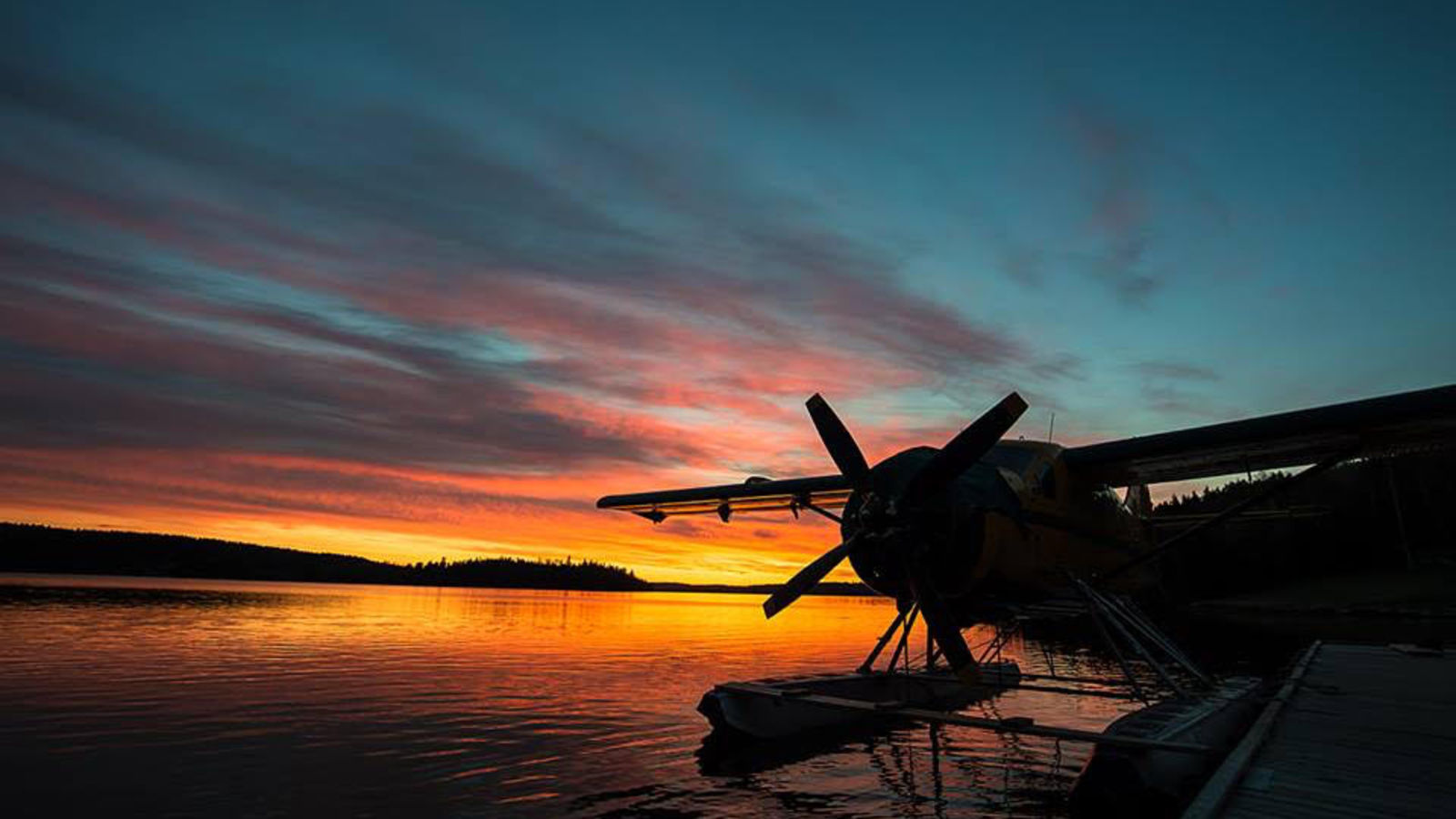This captivating photograph captures the serene ambiance of dusk over a tranquil lake. The main focus is a silhouette of a sea plane, equipped with water landing gear, parked calmly on the still water. To the right, a wooden pier juts quietly into the lake. The expansive sky above is a rich tapestry of sunset colors, transitioning from deep bluish-teal to mesmerizing shades of orange, amber, pink, and hints of purple, adorned with wispy cirrus clouds. The horizon is framed by dark, hilly landmasses, suggesting the presence of distant trees. The reflections of the sunset's glow shimmer softly on the water's surface, enhancing the overall tranquility of the scene. There's an absence of people, lending a peaceful solitude to the image, with only the silhouetted plane, the calm lake, and the embracing sky composing this enchanting dusk tableau.